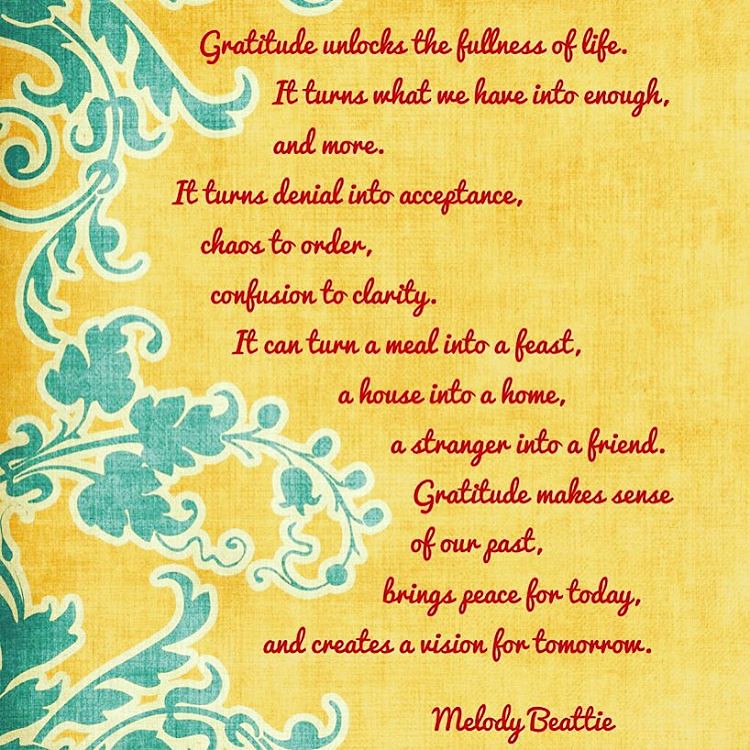The image is a beautifully crafted inspirational card featuring a heartfelt poem by Melody Beattie, centered around the theme of gratitude. The card has a background designed with a yellowed texture and elegant green floral and plant patterns on the left side. The message is rendered in a stunning cursive font in red text, which reads: "Gratitude unlocks the fullness of life. It turns what we have into enough and more. It turns denial into acceptance, chaos into order, confusion into clarity. It can turn a meal into a feast, a house into a home, a stranger into a friend. It can make sense of our past, brings peace for today, and creates a vision for tomorrow. Melody Beattie." The overall color scheme of the card includes red, yellow, and teal accents, all contributing to its uplifting and aesthetically pleasing appearance. This card is designed to encourage appreciation and remind readers of the transformative power of gratitude in their lives.